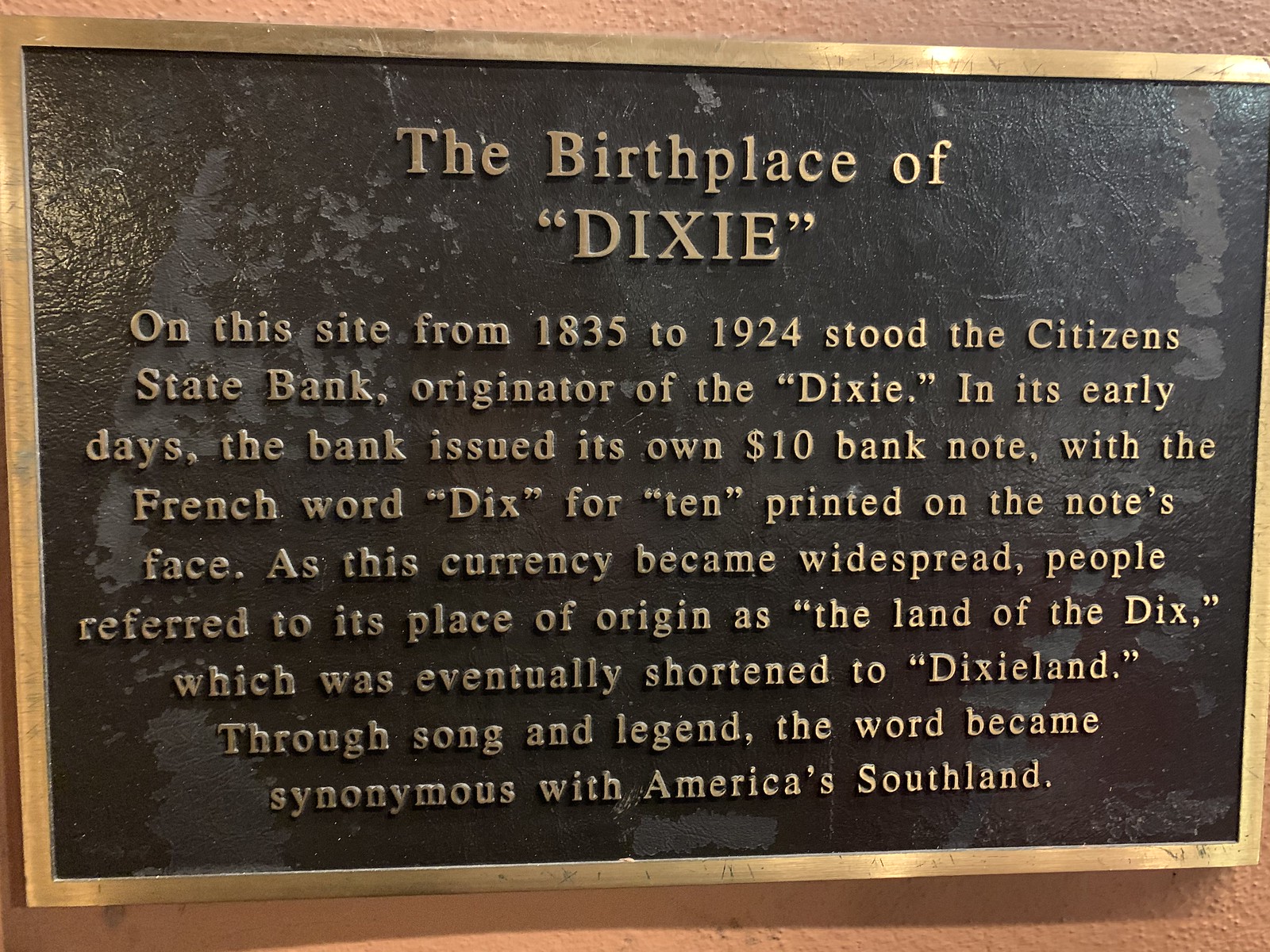The image showcases a historical marker mounted on a peach-colored stucco wall. The marker itself is black with a weathered golden frame and features bronze-engraved text. The rectangular plaque is titled "The Birthplace of Dixie." It explains that from 1835 to 1924, the Citizens State Bank stood at this site and was the originator of the term "Dixie." Initially, the bank issued its own $10 banknote, on which the French word for ten, "DIX," was printed. As this currency became widespread, the area was colloquially referred to as the "Land of the Dix," eventually shortened to "Dixieland." Over time, the term became synonymous with the American Southland through song and legend.